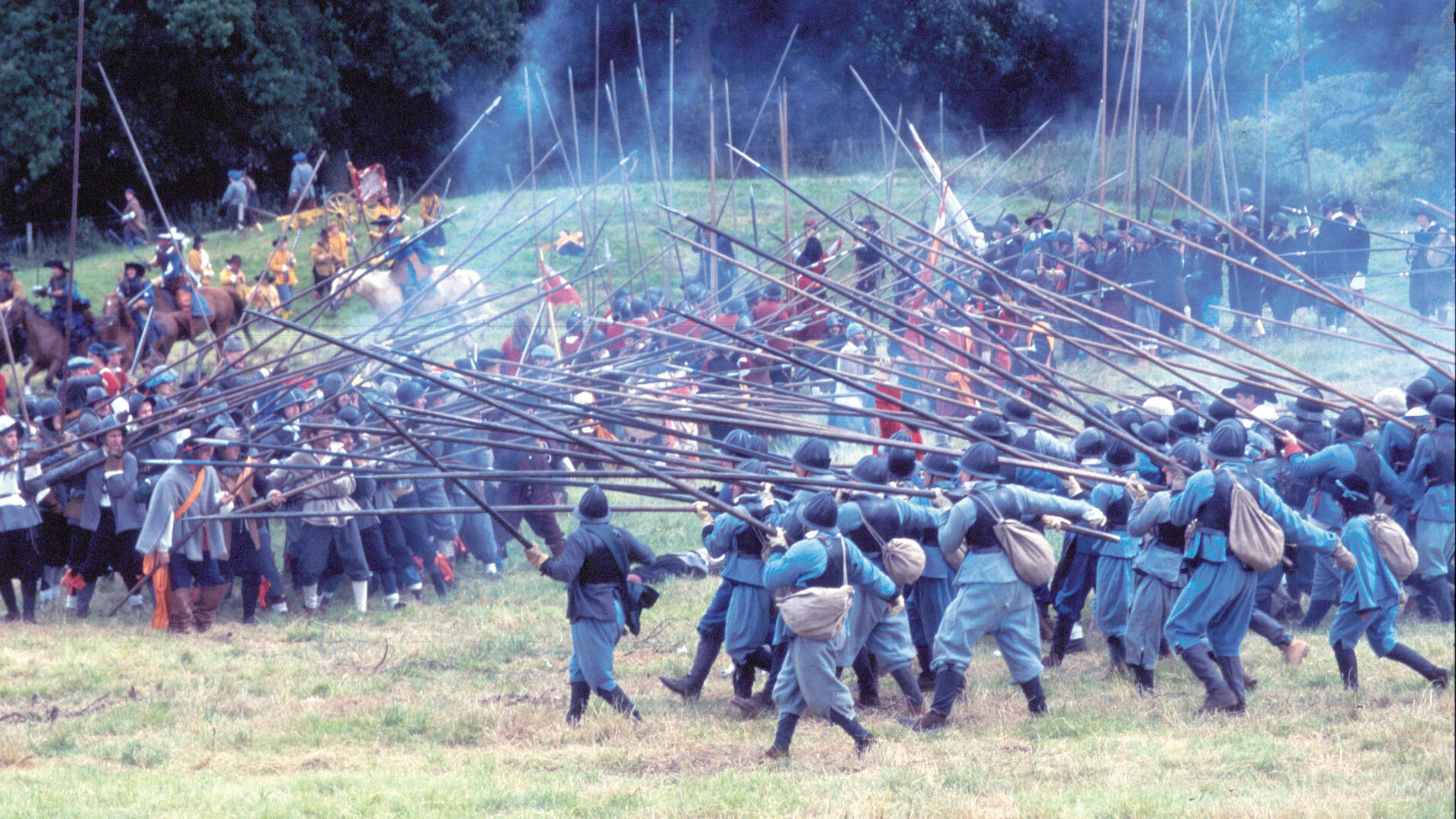The photograph captures an outdoor battle reenactment on a large, partly green and partly brown, grassy field. The scene is vibrant with historical details, showing clusters of people on both the right and left sides of the image. On the right, a group of men is dressed in old-school uniforms with blue pants, blue shirts, black vests, and black boots, carrying brown knapsacks. They hold long, pointed spears poised towards the left. On the left side, more men are dressed in a variety of outfits, including grey jackets and some hints of orange and yellow, also wielding long, pointed poles. Behind this group, a line of riders on horseback is visible, featuring both brown and light-colored horses. Adding to the historical ambiance, smoke, suggestive of gunpowder, wisps upwards from the crowd. The background is framed by a row of trees forming a dense forest line across the top and extending to the right side of the image. The detailed composition and dynamic arrangement of participants vividly evoke a historical battle scene in a lush, natural setting.